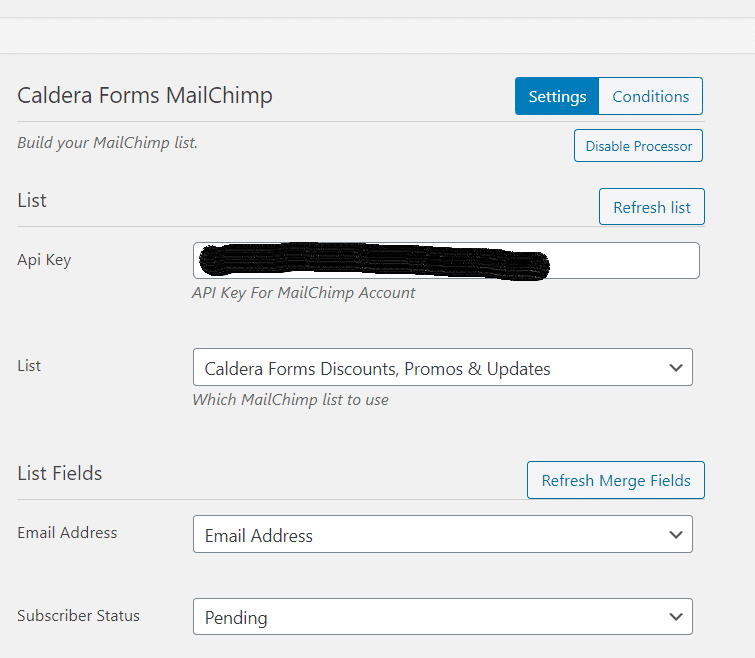**Website Interface for Caldera Forms MailChimp Integration**

The webpage has a clean, all-gray background with navigational options at the top. At the very top, the title "Caldera Forms MailChimp" is prominently displayed. Adjacent to this title, there are two buttons: a blue button with white text labeled "Settings" and a white button with blue text labeled "Conditions."

Beneath the title, in italicized text, the phrase "Build your MailChimp list" is presented. Opposite to this text, on the right side, a checkbox labeled "Disable processor" can be found.

Following this, there is a section labeled "List" with a button next to it that says "Refresh List." Below that, the interface requires an "API Key" for the MailChimp account, with an explanatory note "API key for MailChimp account." The provided key is blacked out for security purposes.

Further down, there's a section titled "Caldera Forms Discounts, Promos, and Updates," indicating the current list selected from a dropdown menu, which allows the user to choose different options. Below this dropdown, italicized text prompts the user to select "Which MailChimp list to use."

Subsequently, in the "List Fields" section, there’s a button in a white box with blue text that says "Refresh Merge Fields." Below this, there's an "Email Address" field with a corresponding dropdown menu. The default selection shows "Email Address" but allows for other choices. Finally, another dropdown menu for "Subscriber Status" shows the status as "Pending," with options to select different statuses.